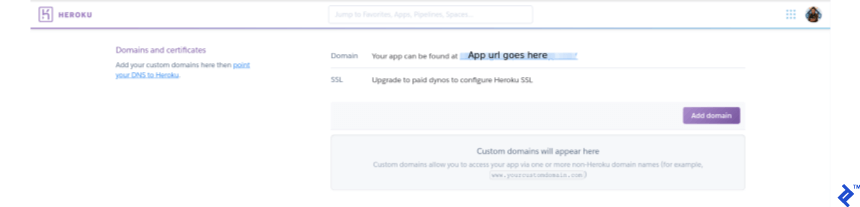This image is a detailed screenshot of a web page from Heroku. At the top left corner, the Heroku logo and name are prominently displayed. The top center features a browser address bar, while the top right corner includes a profile picture. The website content is divided into two main sections.

On the left, in purple letters, is the title "Domains and Certificates." Below this title, there is a hyperlink titled "Point your DNS to Heroku." 

To the right of this section lies a chart. The first entry in the chart is "Domain," followed by the statement "Your app can be found at app URL goes here." Below this, the next entry is "SSL," with the instruction "Upgrade to paid dynos to configure Heroku SSL" to the right. Toward the far right side, there is a purple button labeled "Add Domain."

Additionally, there is a small box with the title "Custom Domains" indicating that custom domains will be shown there. In the bottom right corner, there appears to be a trademark symbol next to an image resembling a tilted blue chair.